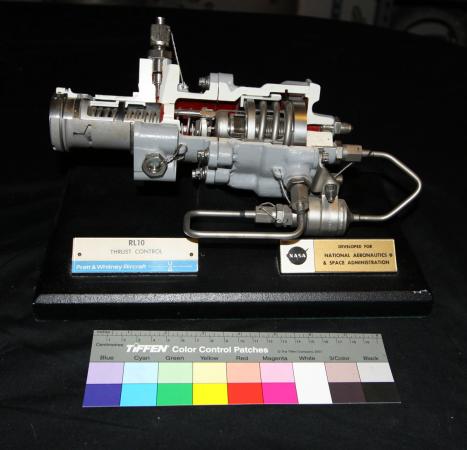The image showcases a detailed NASA thrust control device, prominently displayed against a black fabric and wood backdrop. The metallic, tubular device features a cutaway section that reveals intricate inner workings, including coils and springs, providing a glimpse into its sophisticated engineering. Adjacent to the device is a placard labeled "RL-20 Thrust Control," along with another placard that reads, "NASA - National Aeronautics and Space Administration." In the foreground, a Tiffin control patch with various colors, including blue, cyan, green, yellow, red, magenta, black, and white, is visible. The colors are presented in small square boxes, with each color represented in both lighter and darker shades. The entire display is meticulously arranged, emphasizing the complexity and precision of the NASA technology.